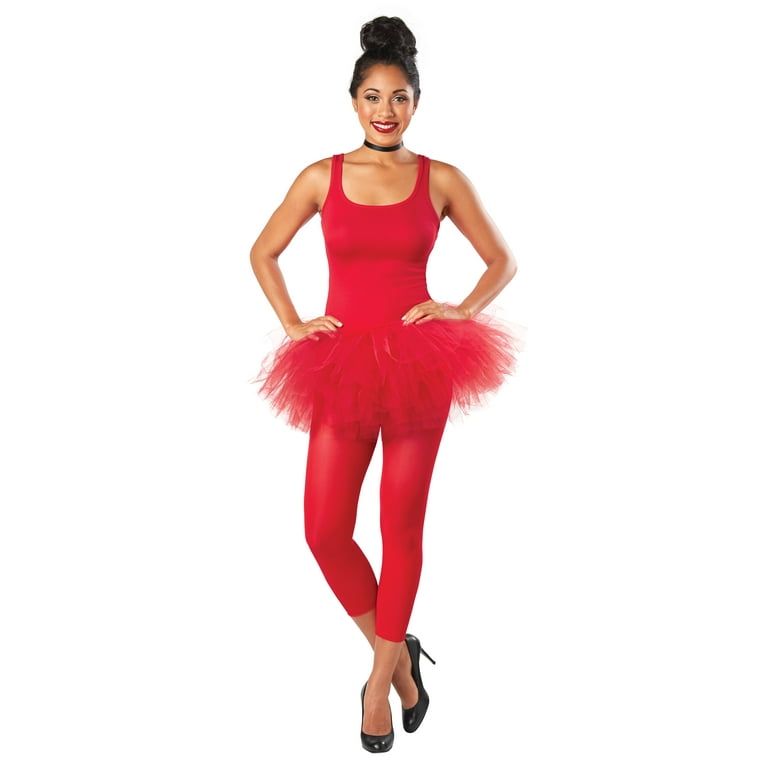In this detailed photograph, a young woman poses confidently against a stark white backdrop. She wears a striking red, almost pinkish, ballerina tutu that includes both a frilly skirt and a body-hugging leotard, extending sleeveless from her shoulders to her mid-calf. Complementing her outfit are black high-heeled shoes which emphasize her poised stance. Her right leg is elegantly crossed behind her left, with her toe to the ground and heel lifted. 

The woman's dark hair is neatly styled in a ballet bun atop her head, and she sports a black choker necklace that accentuates her graceful neck. Her makeup includes bright red lipstick that vividly matches her tutu, contrasting beautifully with her darker complexion. Her brown eyes are wide and lively, and her bright white teeth frame a radiant smile. Adding to her polished appearance, her nails seem to be painted in a pale white color. With hands confidently resting on her hips, she exudes a poised elegance, making it likely she is posing for a ballet portrait.